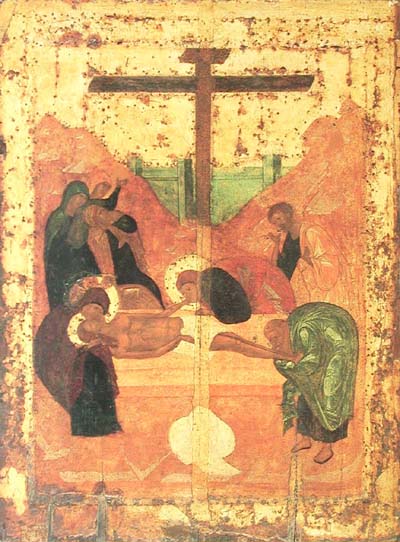This is a tall, rectangular, religious painting with an aged and faded appearance. The background is primarily yellow, covered in burnt orange, brown speckles, and splotches, giving it an antique feel. Central to the painting is a large, dark brown cross situated at the top, which extends down towards a greenish fence-like structure. In the foreground, there is a scene depicting Jesus, characterized by his dark orange skin and a white cloth around his waist, lying on a slab or bed. Surrounding him are six figures draped in thick, heavy robes. To the left, a woman is tenderly holding Jesus' head in her lap, while to the right, a man kisses his feet, and another woman appears to touch or kiss his arm. Additional figures are positioned behind these primary characters, some with arms outstretched, seemingly gesturing towards the cross. The color palette of the painting features muted, earthy tones of yellow, orange, red, and brown, adding to its venerable aesthetic.